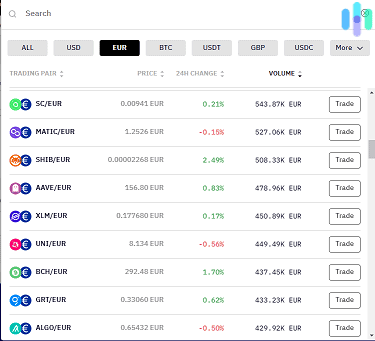In this image, we see a detailed view of a stock trading website interface. At the top, there is a search bar for quick navigation. Directly below the search bar, there is a horizontal row of rectangular icons, each representing different currencies or categories. From left to right, these are labeled: "All," "USD," "EUR," "BTC," "USDT," "GBP," "USDC," and a final icon labeled "More" accompanied by a down arrow. The "EUR" icon is prominently highlighted in black, while the remaining icons are displayed in light grey, indicating the currently selected currency filter.

Beneath these icons, the interface lists various stock trading pairs, each accompanied by a set of details. For each pair, the image shows the current price, the 24-hour change expressed as a percentage (with increases highlighted in green and decreases in red), and the trading volume. Additionally, there is a "Trade" button available next to each trading pair for quick access to trading actions.

The trading pairs are also indicated by names and associated with small circular icons, which presumably represent the respective currencies or assets in each pair. This meticulous layout facilitates easy tracking and trading of various currency pairs on the platform.